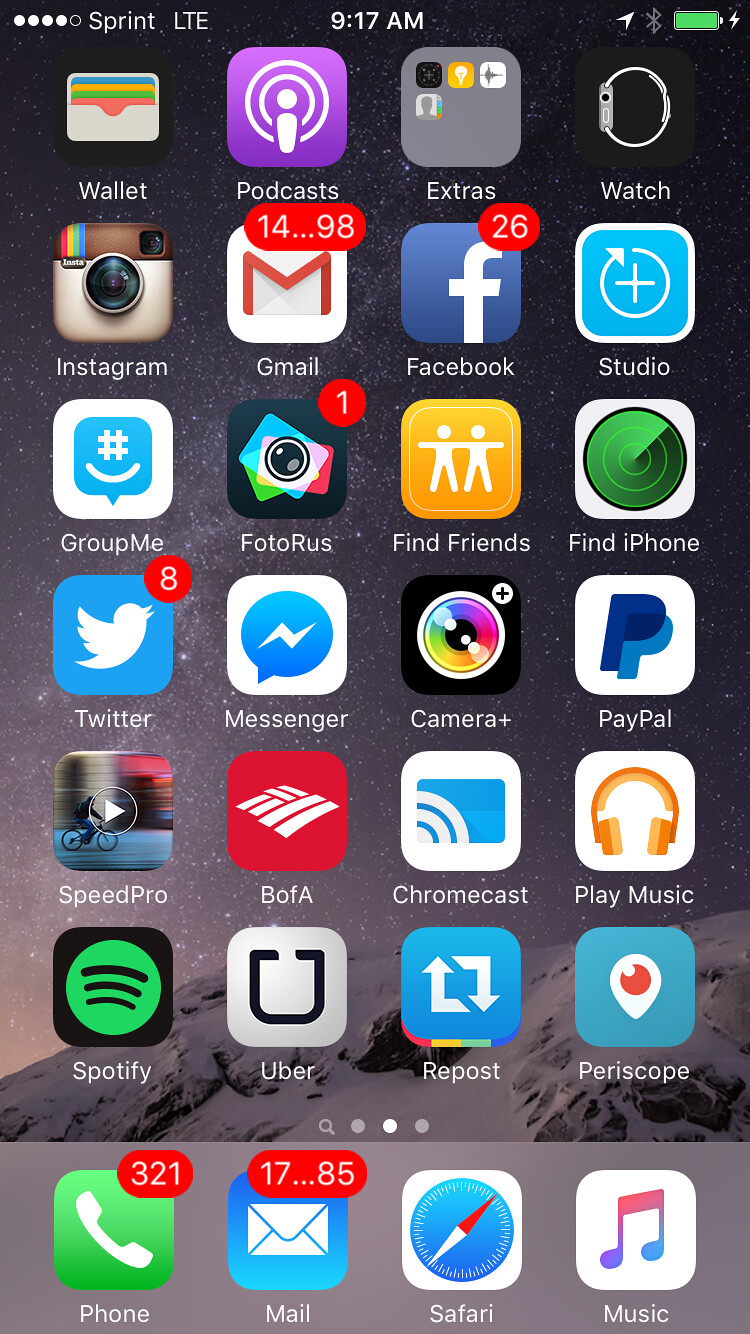This image appears to be a screenshot from a mobile phone. The background features a serene night sky and a range of snowy mountains. At the top of the screen, the status bar shows network details with "Sprint LTE" service, the current time of 9:17 AM, and a fully charged battery indicator.

The home screen displays various app icons sorted across multiple rows. Notably, the phone app at the bottom has 321 notifications, while the Mail app shows an overwhelming 17,085 unread messages. In the same dock, the Safari web browser and a music app are also present.

The rest of the home screen is populated with a collection of apps including Spotify, Uber, Repost, Periscope, SpeedPro, Wofa, Chromecast, Google Play Music, Twitter, Messenger, Camera, PayPal, GroupMe, PhotoPlus, Find Friends, Find iPhone, Instagram, Gmail, Facebook, YouTube Studio, Wallet, Podcast Extras, and the Watch app. Each icon is clearly visible against the aesthetically pleasing night sky and mountain backdrop.